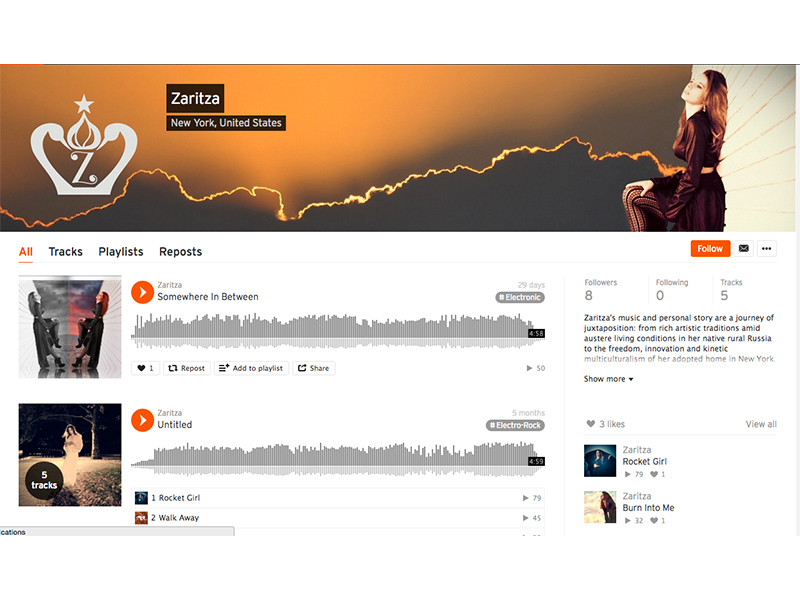The image shows a detailed view of a computer screen displaying information about the singer Tsaritsa. The top section features Tsaritsa herself or her album cover. She is a Caucasian woman with fair skin and reddish hair, dressed in dark clothing that appears to be a dress with intricate designs. Her outfit includes stockings or pants with visible lines. A striking visual element is a lightning streak originating from one side of her figure, crossing the entire image. A crown symbol with the letter "Z" is also prominent.

The screen displays "Tsaritsa, New York, United States", highlighting her location. The interface shows a psychedelic album cover, accompanied by another image of her wearing a white dress. This section lists five tracks, including "Rocket Girl" and "Number Two, Walk Away". The profile indicates that she has eight followers, is following no one, and has five tracks in her collection.

A detailed narrative describes Tsaritsa's musical and personal journey, contrasting her rich artistic roots in rural Russia with the dynamic and culturally diverse environment of New York. Her music, which blends electronic and electro-rock genres, reflects this unique fusion of influences. An orange "Follow" button and options to play her music are also present on the screen, inviting listeners to explore her work further.